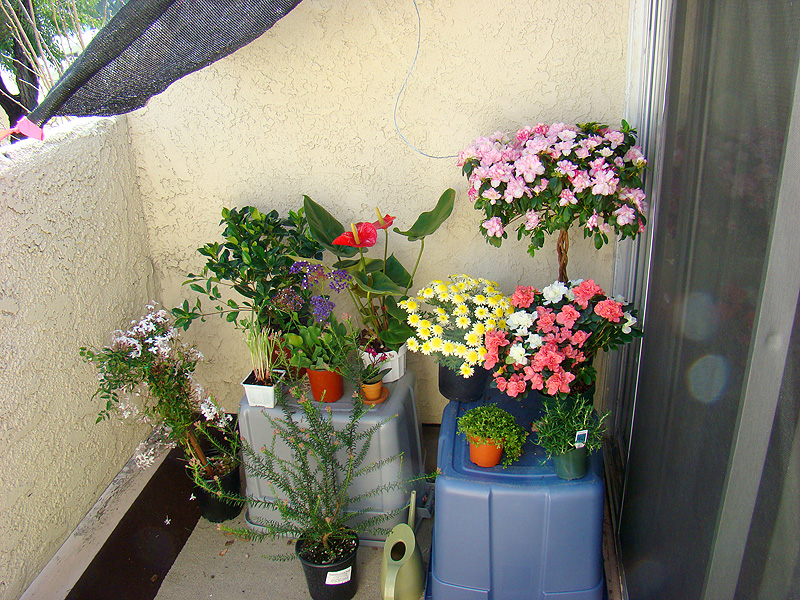The image captures a cozy, small patio area outside an apartment, bathed in bright sunlight. This patio, which extends about three to four feet from the sliding glass door visible on the right, has low cement-textured walls around it. In the foreground, there are two plastic storage totes turned upside down to function as tables. The blue tote on the right holds five potted plants, three of which are flowering in shades of yellow, pink, and a brighter pink. On the left, the gray tote supports six potted plants, with additional plants arranged at its base. Various plant species, such as anthurium, a braided tree with pink blossoms, and possibly a zizi plant, add vibrant greenery to the space. The patio is covered with a screen filtering the sunlight, ensuring the plants receive sufficient light without getting scorched. The combination of the totes and numerous plants transforms this tiny exterior into a lush, colorful garden nook.